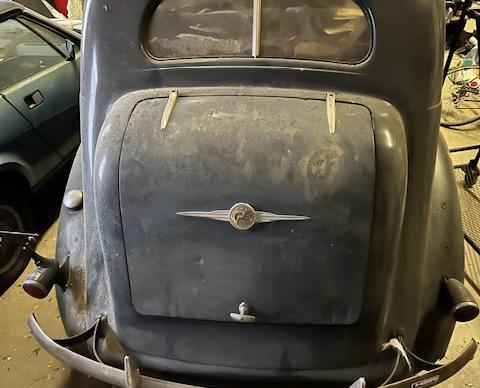The image is a color photograph capturing a close-up of the back end of an antique car, likely from the 1930s or 1940s, surrounded by muted colors. The car, possibly a Studebaker, is dark gray with patches of rust revealing the underlying metal. It features a silver curved bumper, gray metal hinges, a small handle at the trunk, and dual exhaust pipes. The taillights are visible, and a narrow rounded rear window with a silver bar runs through the middle. In the background, to the left, there is a glimpse of a more modern car, possibly from the 1970s or 1980s, painted green. The scene appears to be set in a junkyard or possibly a private collection area, with hints of additional vehicles and a bike wheel partially seen on the ground, indicating an outdoor environment during the day.